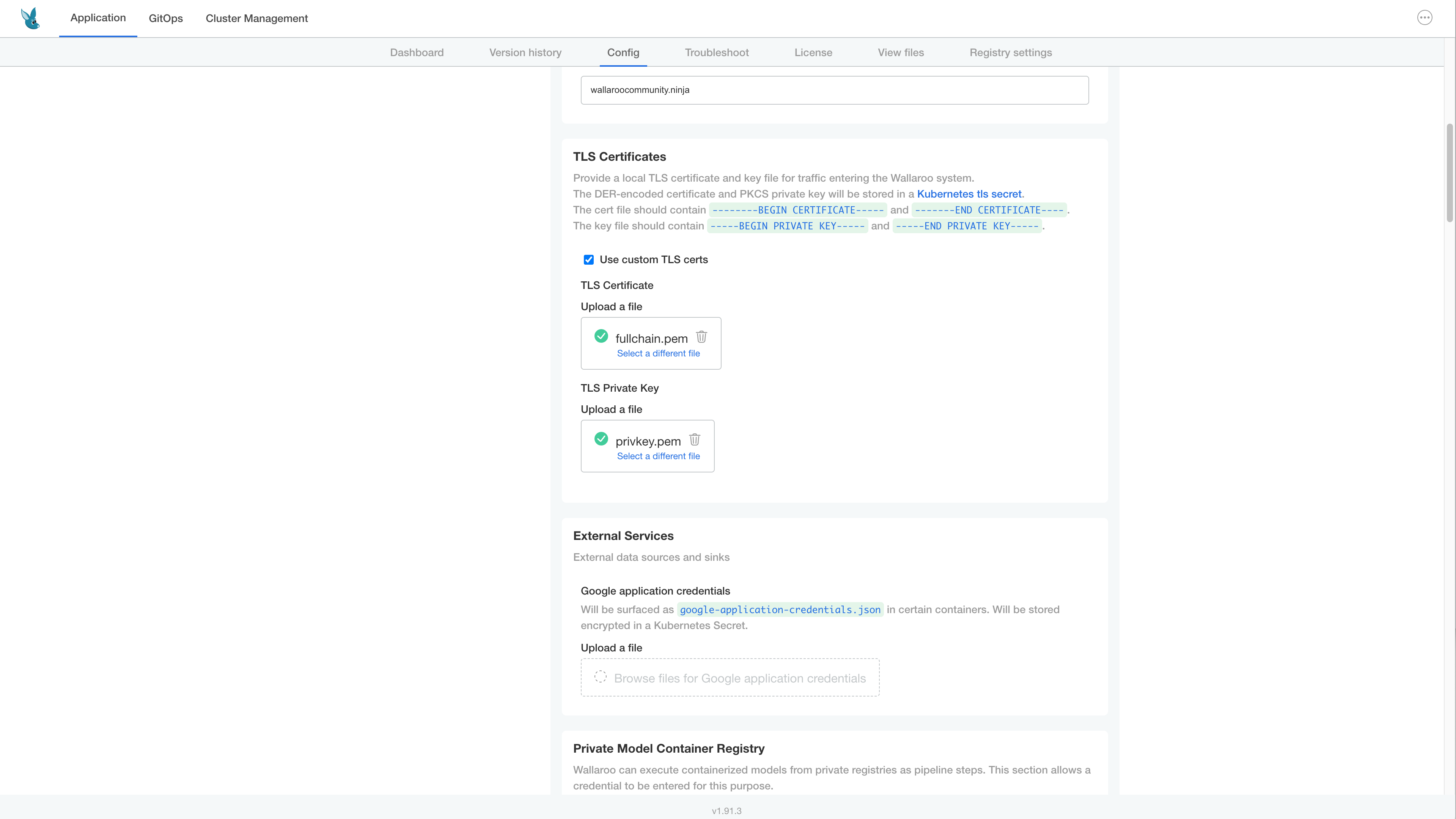This image is a cropped screenshot of a configuration panel on a web page. In the top-left corner, there's a small, blue icon resembling an insect. To the right of this icon, the text reads "Application." Below, it lists "GitOps and Cluster Management," with the "Application" section currently selected and indicated by a blue underline.

Directly underneath these categories, a gray navigation bar centered on the screen displays various options: Dashboard, Version, Config, Troubleshoot, License, View Sites, and Settings. The "Config" option is selected, which causes a detailed configuration panel to appear.

At the top of the configuration panel, there is a text box. Below this, a white box labeled "TLS Certificates" contains highlighted text descriptions: "Begin Certificate," "End Certificate," "Begin Private Key," and "End Private Key." All these options are highlighted in blue.

Further down, there's a checkbox labeled "Use Custom TLS Certs," which is selected. Beneath this, the labels "TLS Certificate" and "Upload a File" indicate where files can be uploaded. A file has been successfully uploaded, as shown by a green check mark to the left of the file name.

Under this, the section for "TLS Private Key" also has an "Upload a File" option. It shows that a file has been uploaded, indicated by a green circle with a white check mark next to it. This detailed caption provides a clear and thorough description of the configuration panel's layout and current selections.